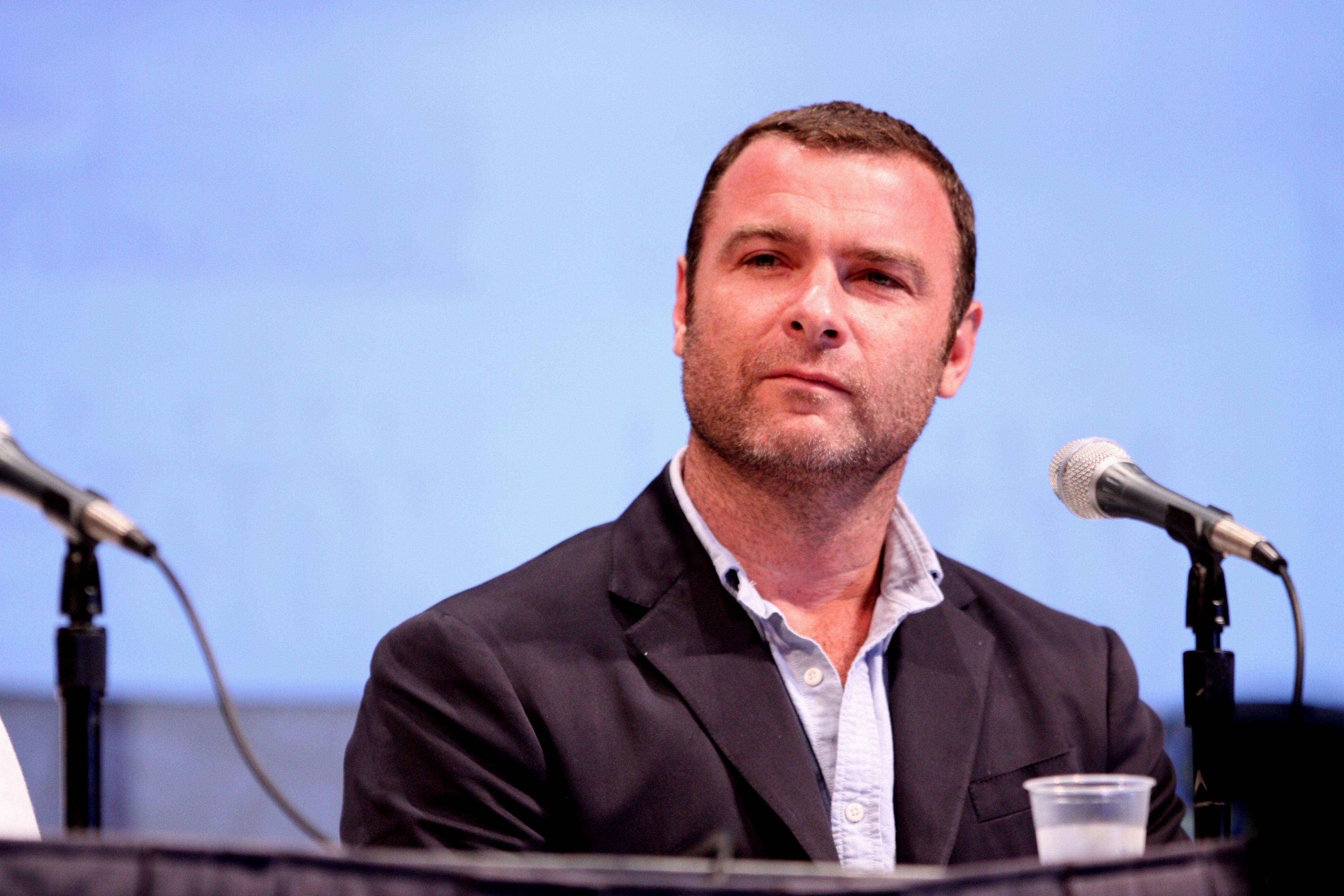The image features a man seated at a panel, likely during a convention such as Comic-Con. He has a ruddy complexion, very short, dark brown hair, and a lightly stubbled beard indicating a few days without shaving. His face is quite round, and his eyes are slightly squinted as he appears to be listening attentively or deep in thought, directed towards someone to his right. He is dressed in a casual, slightly wrinkled black jacket, possibly felt-like in material, over a light blue button-up shirt with white buttons. In front of him is a traditional silver microphone on a black stand, as well as a plastic cup with some water inside. The background is a light blue wall, adding a calm and focused atmosphere to the setting. To his left, another microphone is visible but positioned just out of sight of the adjacent person. The image captures him from the head and shoulders down to about halfway down his arm, with the table rim also visible in front of him.